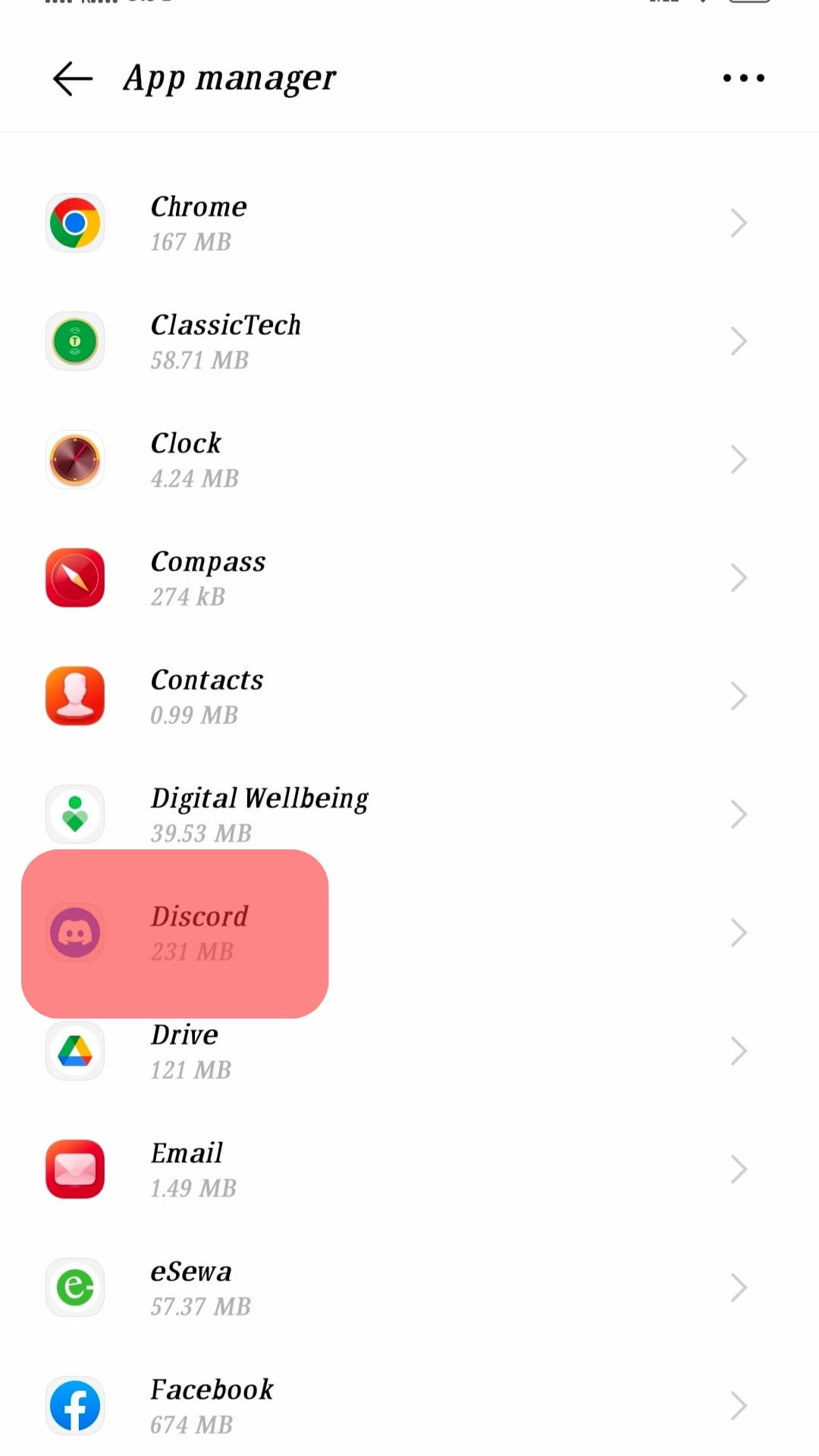This image is a detailed screenshot taken from a smartphone, showcasing the "App Manager" section. The title "App Manager" is displayed in black italicized font at the top left corner, accompanied by a left-pointing arrow, likely indicating a back button. 

The background is predominantly white, providing a clean and clear display of a lengthy list of app icons and names. The icons are aligned to the left, with the app names slightly more centered. To the right of each app name, small gray arrow icons are visible, indicating expandable menu options.

The listed apps include Chrome, Classic Tech, Compass, Clock, Contacts, Digital Wellbeing, Discord, Drive, Email, eSua, and Facebook. Notably, the Discord app entry is highlighted with a light red rectangular box around both its icon and name, drawing attention to it. Below each app name, storage information is detailed in megabytes (MB).

In the upper right corner of the screen, there are three vertical dots, hinting at additional settings or menu options. This well-organized interface offers a comprehensive view of the various apps installed on the device, along with their respective storage usage.